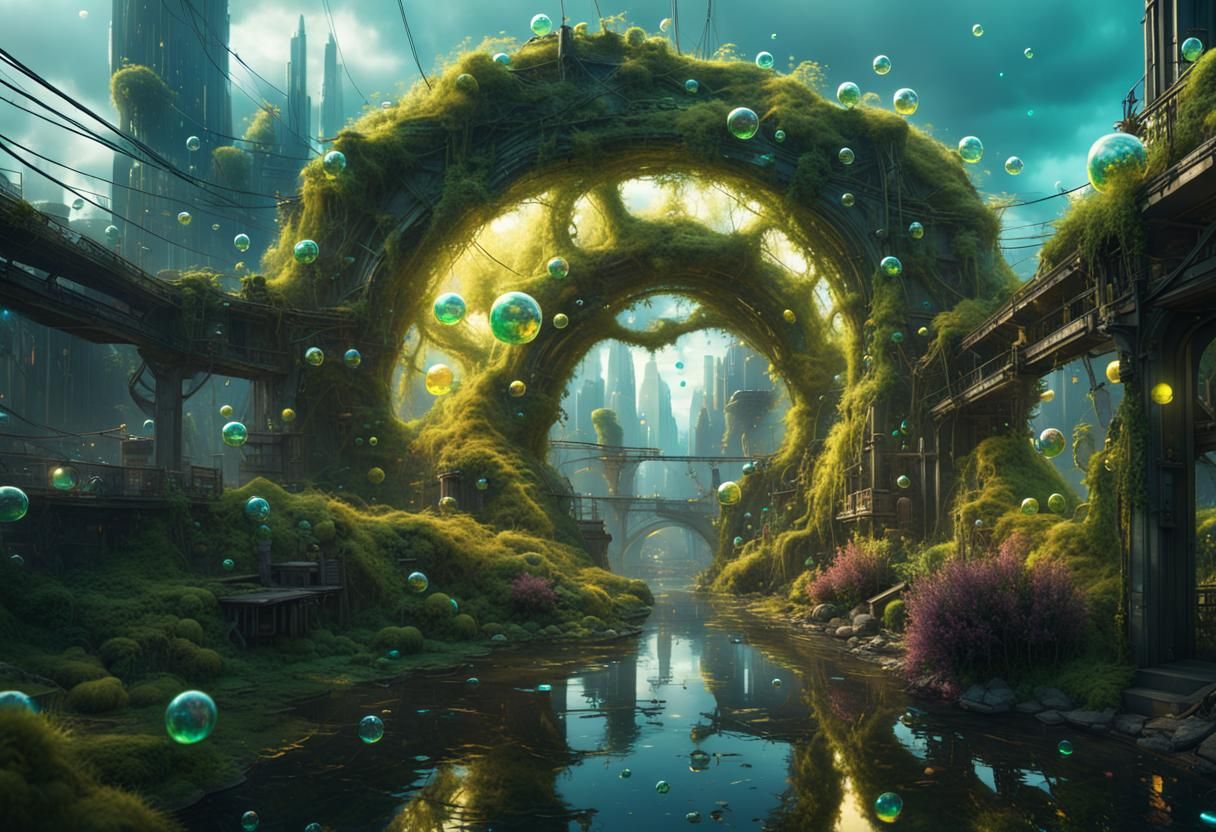In this remarkably detailed AI-generated scene, a fantastical waterway stretches into the distance, its calm, dark waters bordered by semi-circular structures covered in lush, lime-green moss. These structures, resembling ancient stone rings, create a tunnel-like pathway that guides the eye toward a distant vanishing point. Floating throughout the vivid blue-green sky are jewel-like bubbles, predominantly clear with hues of jade green and occasional yellow, varying in size from baseballs to basketballs.

On either side of the serene stream or creek, banks flourish with moss and a variety of plants, including distinct reddish and purple bushes. In the upper left background, towering, futuristic skyscrapers rise, their heights far exceeding those of modern cities. Sunlight filters from behind these imposing buildings, casting a glow across the scene. To the right, additional structures stretch into the distance, adding to the dreamlike quality of this panoramic view. Bridging the waterway at intervals are moss-covered arcs, enhancing the scene's mystique and the enchantment of this otherworldly, almost realistic depiction.